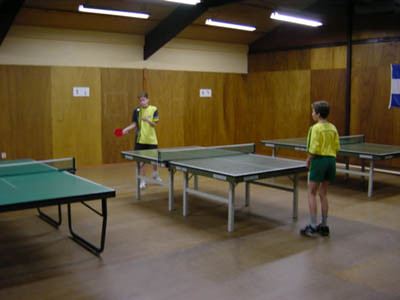In this vibrant, color photograph, an indoor recreation room features prominently, characterized by its brown wood-paneled walls and overhead fluorescent ceiling lights. Three ping pong tables with green tops and white markings are neatly aligned in the center of the room. The tables vary slightly in design, with one table sporting dark-colored legs, contrasting with the two tables that have white legs.

At the center table, two teenage boys are deeply engrossed in a lively ping pong match. Both teenagers, who have brown hair, are outfitted identically in yellow t-shirts with green accents and green shorts. The teenager on the left, seen mid-game with his red paddle held to the side, wears white socks and white sneakers. His opponent, standing at the forefront of the photograph, also sports white socks but pairs them with dark sneakers.

Notably, a blue and white flag hangs in the corner of the room, adding a splash of color to the warm, wood-paneled setting. The room’s distinct combination of elements—wood paneling, fluorescent lighting, and athletic activity—captures a lively, engaging atmosphere.